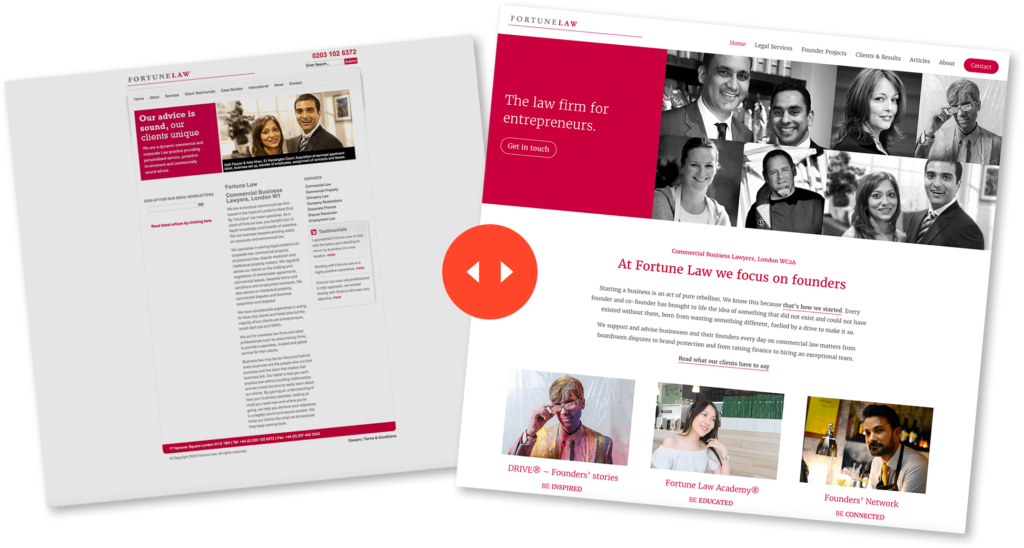The image comprises two overlapping screenshots, with the right screenshot appearing bright and centrally focused, while the left is grayed out and less discernible. 

**Left Screenshot:**

- **Header:** Displays "Fortune Law" with "Fortune" in gray and "Law" in red, underscored by a line. 
- **Top Row:** Contains a small, illegible phone number.
- **Topics:** Below the header, several hard-to-read topics are listed.
- **Red Panel:** Features white text stating "Our advice is sound, our clients are unique" followed by additional writing.
- **Imagery:** Displays a picture of a man and a woman in business casual attire with a caption beneath their photo.
- **Content:** An article with multiple paragraphs appears at the bottom.

**Right Screenshot:**

- **Header:** Similar to the left, showing "Fortune Law" with "Fortune" in gray and "Law" in red. 
- **Navigation:** To the right of the header, it lists "Home," "Legal Services," "Clients and Results," "Articles About," and a red "Contact" button.
- **Red Text Box:** States "The law firm for entrepreneurs" in white letters, with a "Get in touch" button underneath.
- **Imagery:** Features a group photo of eight individuals, consisting of five men and three women.
- **Commercial Business Lawyers Section:** Includes red text that reads "Commercial Business Lawyers."
- **Content:** Highlights "At Fortune Law, we focus on founders" with a brief paragraph beneath it.
- **Team Section:** Contains pictures of three different individuals with their names and clickable items.

This detailed caption provides a comprehensive view of the overlapping screenshots, emphasizing the central features and text to offer clarity and context.